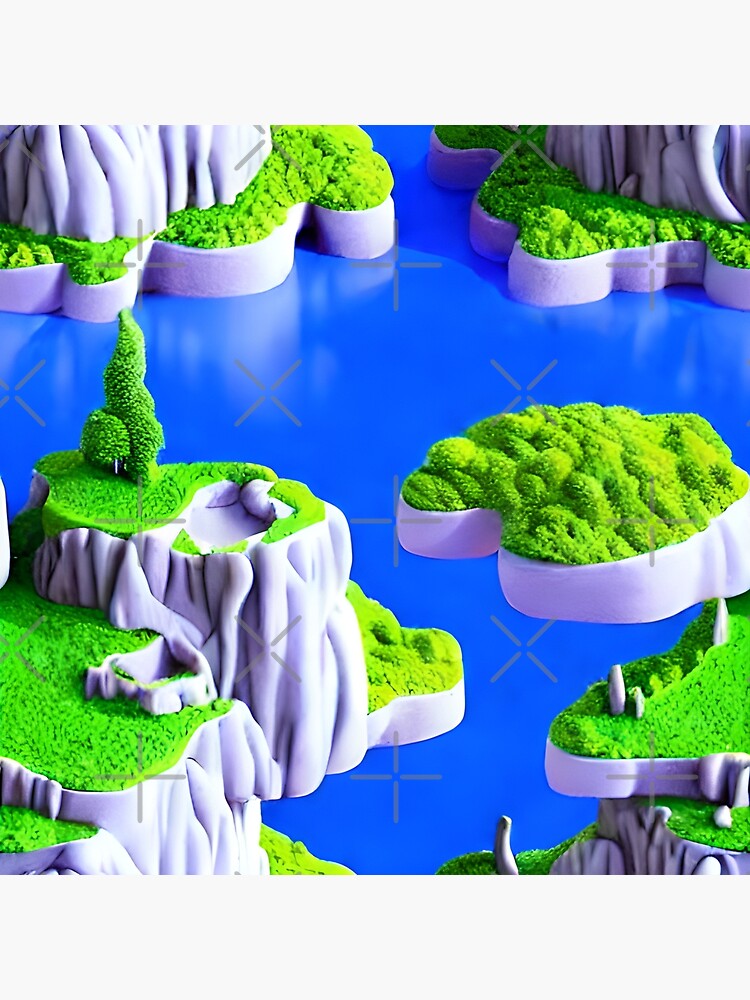The image appears to be a detailed CGI or cartoon rendition featuring a vibrant electric blue body of water interspersed with numerous small land masses, islands, and rock outcroppings. These formations range from four to eight inches in height and are depicted in light gray, adorned with lush, vibrant green vegetation, which includes both ground cover and trees. The landscape bears an almost miniature model-like appearance, reminiscent of pieces one might use to set up a model village, with clear, stony bases and greenery atop. Some of the rock formations are prominently covered in a mossy or low-lying grass-like material, while others boast small trees. The image also includes sparkling effects in the water, represented by gray X’s, enhancing its whimsical, digital aesthetic. There are at least two larger pieces in the background whose tops are not visible, adding depth and a sense of scale to the scene. This detailed depiction blurs the line between a still from a video game and a well-crafted digital model, with its intricate, yet somewhat indistinct, artistic quality.